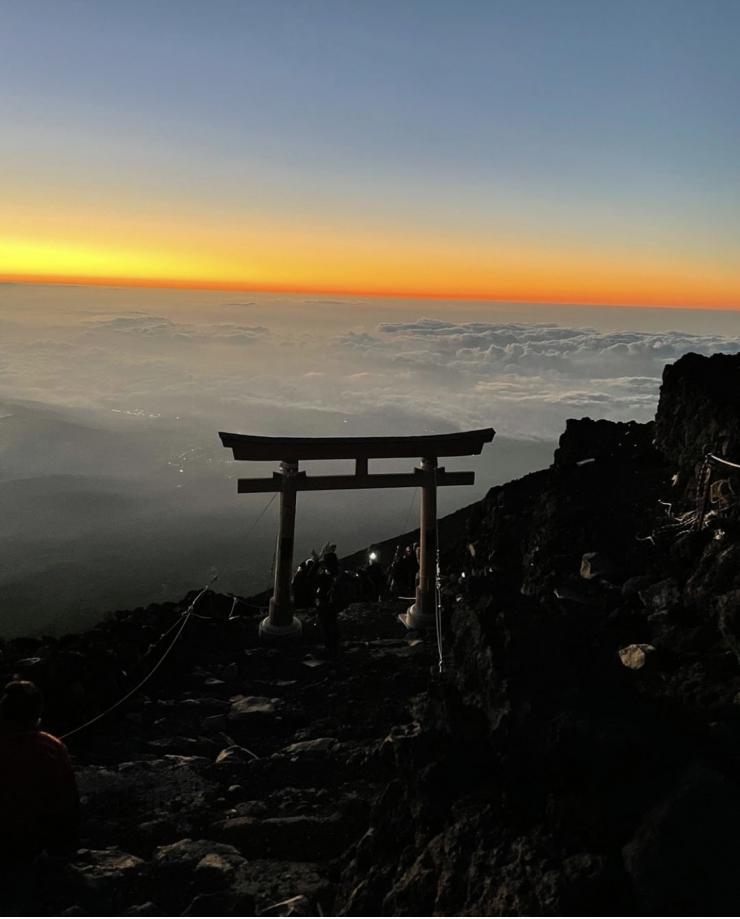Perched atop a high mountain, this striking photograph captures an expansive valley cloaked in dense clouds that obscure the earth below. Dominated by a dramatic sky transitioning from intense orange and deep red hues at the horizon to lighter yellows and finally a fading blue higher up, the image suggests the serene beauty of either a sunset or sunrise. In the dimly-lit foreground, dark and rocky terrain envelops the scene, accentuated by a traditional Japanese torii gate standing sentinel with its two tall pillars and a horizontal spar. Silhouetted figures form a crowd nearby, their details lost in shadows. This picturesque landscape embodies a breathtaking blend of natural tranquility and cultural touchpoints, inviting viewers to explore its mystique.